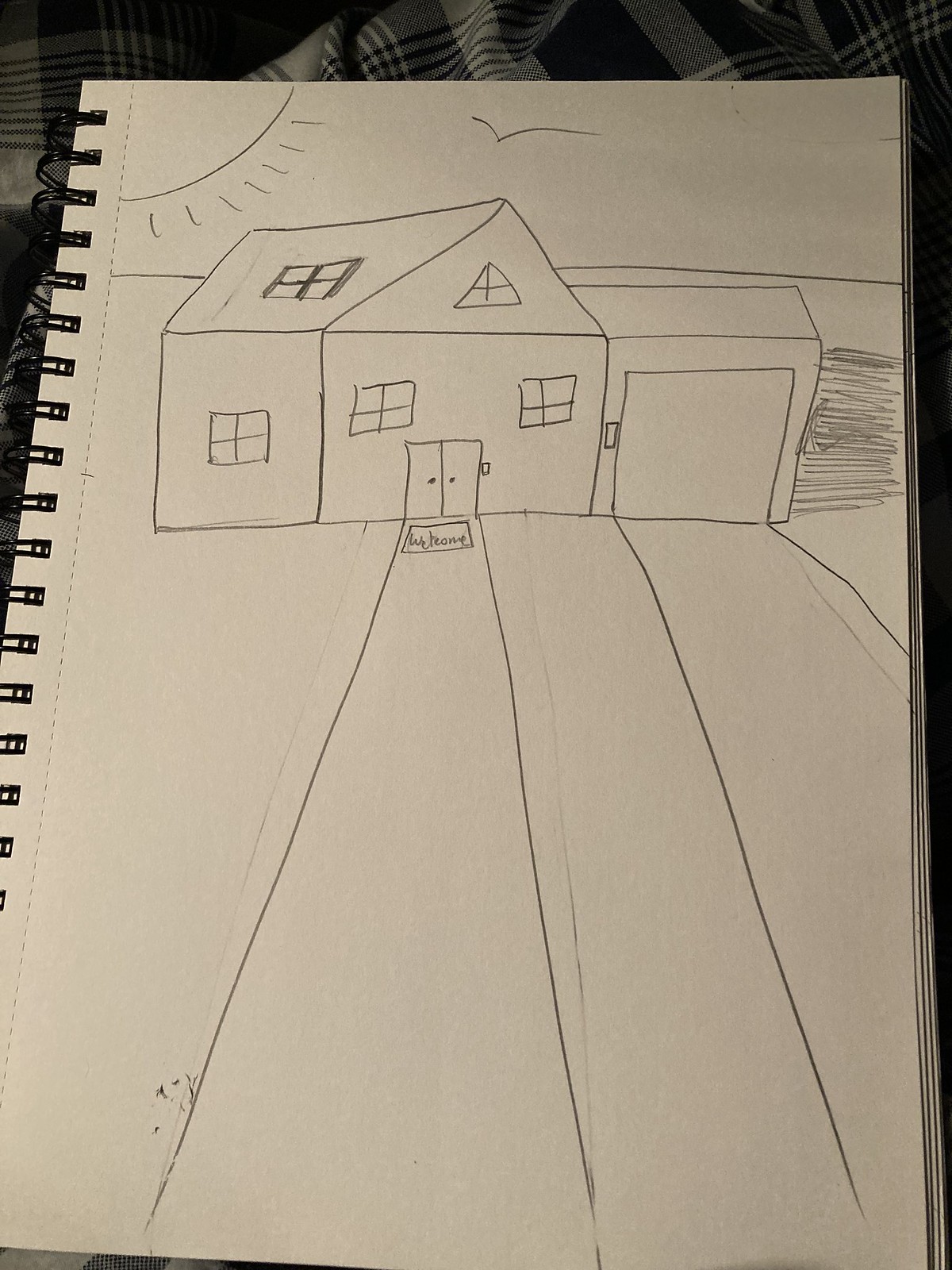This photo captures a sketch on a white, plain-paper notebook with black spiral binding. The drawing appears to be rudimentary, resembling the work of a child. The sketch depicts a house with a square front and a pitched gable roof. There are windows on the sides and front, as well as an unusual window on the roof. The front features a double door with a welcome mat and a long sidewalk leading up to it. Adjacent to the house, a garage is drawn. In the sky above, a sun and a bird are depicted, adding a whimsical touch to the scene.